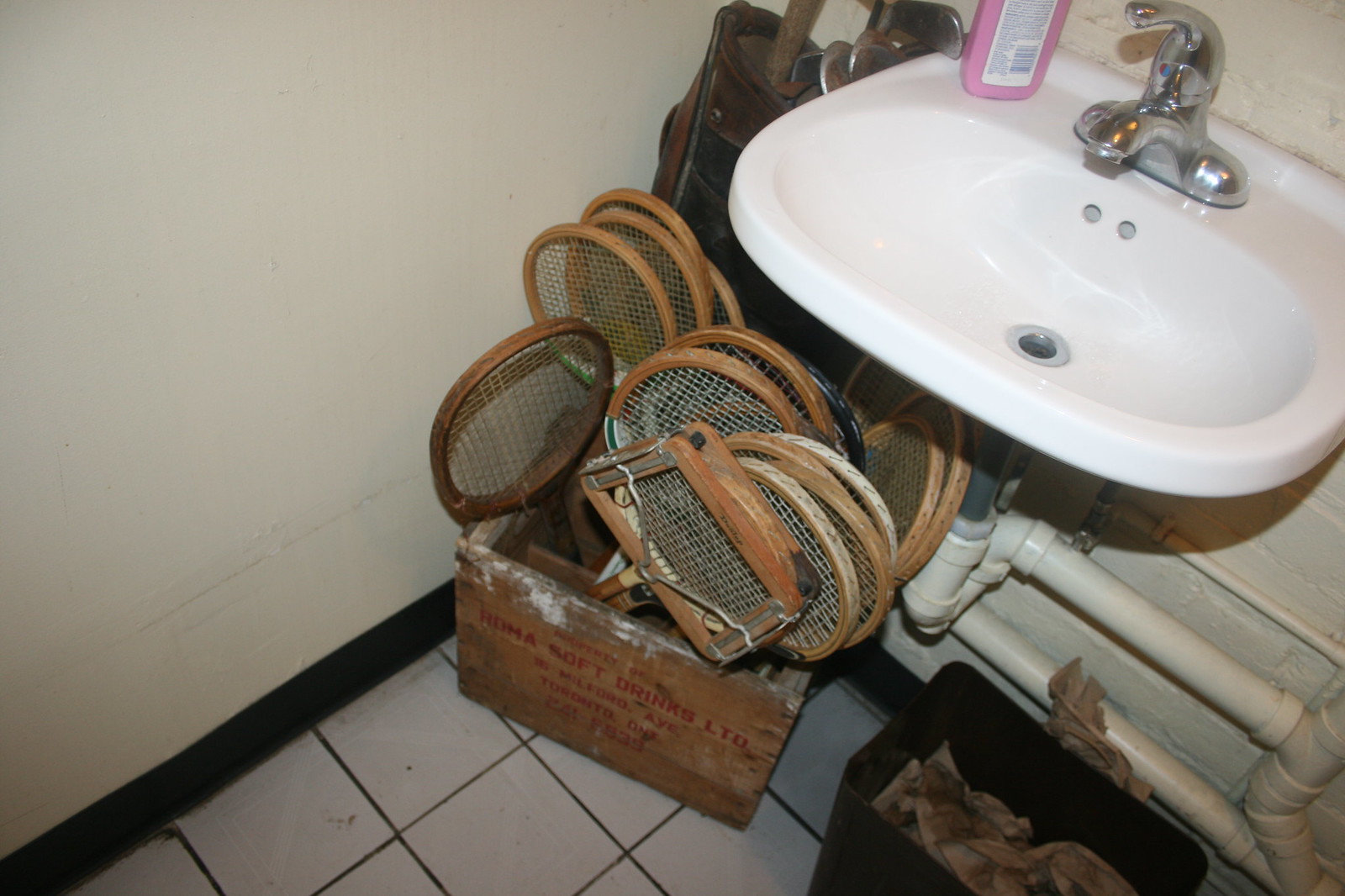The photograph depicts a neat and clean room with an old-style white porcelain sink mounted on the wall, lacking a vanity. The exposed plumbing underneath the sink is painted eggshell white, matching the wall's color. The faucet is a single-handled, chrome-finished type with a pull knob and color-coded indicators for hot (red) and cold (blue) water. To the left of the faucet, there is a pink bottle with its back label visible.

The floor is covered with square white tiles featuring black grout lines. Against the wall, beneath the sink, is a wooden crate marked with the text "Roma Soft Drinks LTD" in black. The crate houses around ten vintage wooden tennis rackets with their heads sticking out. One racket appears to be synthetic, and another has a distinctly square shape. Behind the crate, barely visible, is a dark brown golf bag filled with old golf clubs.

To the right of the crate, there is a dark brown plastic bin containing slightly wet, light brown paper towels. The entire room has a slightly dated yet orderly appearance, with a focus on the various sporting equipment and the functional, exposed-pipe sink setup.